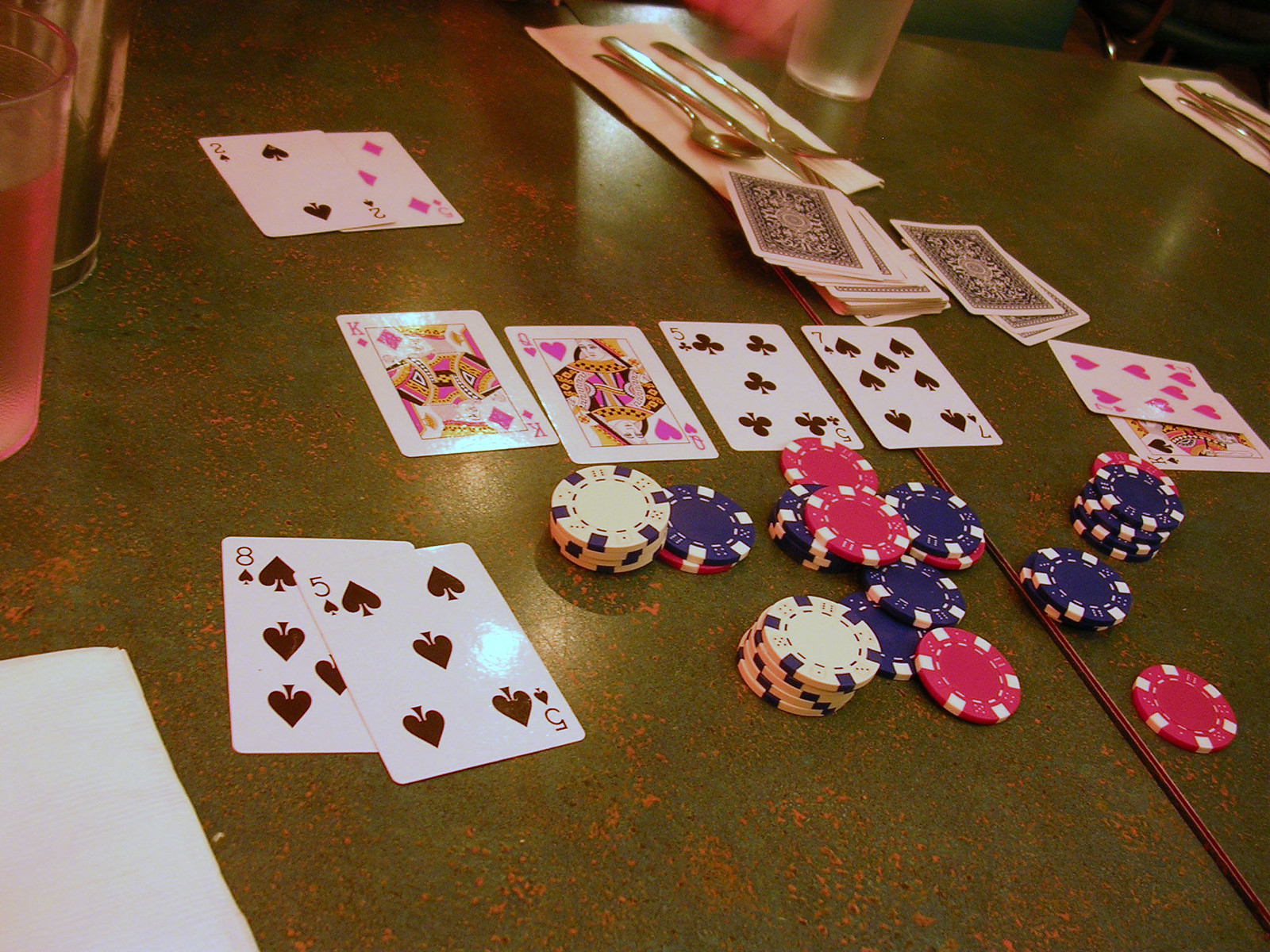The photograph showcases a poker table that features a blend of green and brown hues. At the center of the table, four playing cards are prominently displayed: the King of Diamonds, Queen of Hearts, Five of Clubs, and Seven of Spades. Arranged in front of these cards are neatly stacked poker chips in blue, red, and white.

To the left of the central cards, an Eight of Spades and a Five of Spades are laid out. On the right, there's a King of Spades and a Seven of Hearts. Positioned behind the central quartet, a Five of Diamonds and a Two of Spades are revealed face-up. 

The left side of the image features two cups, one pink and one clear. A napkin lies in the bottom left corner. Additionally, two decks of cards are stacked face-down to the right and slightly above the central cards. In front of these decks, a napkin with a fork, knife, spoon, and another clear cup is neatly arranged. This detailed arrangement and the diverse elements on the table capture the essence of an ongoing poker game.